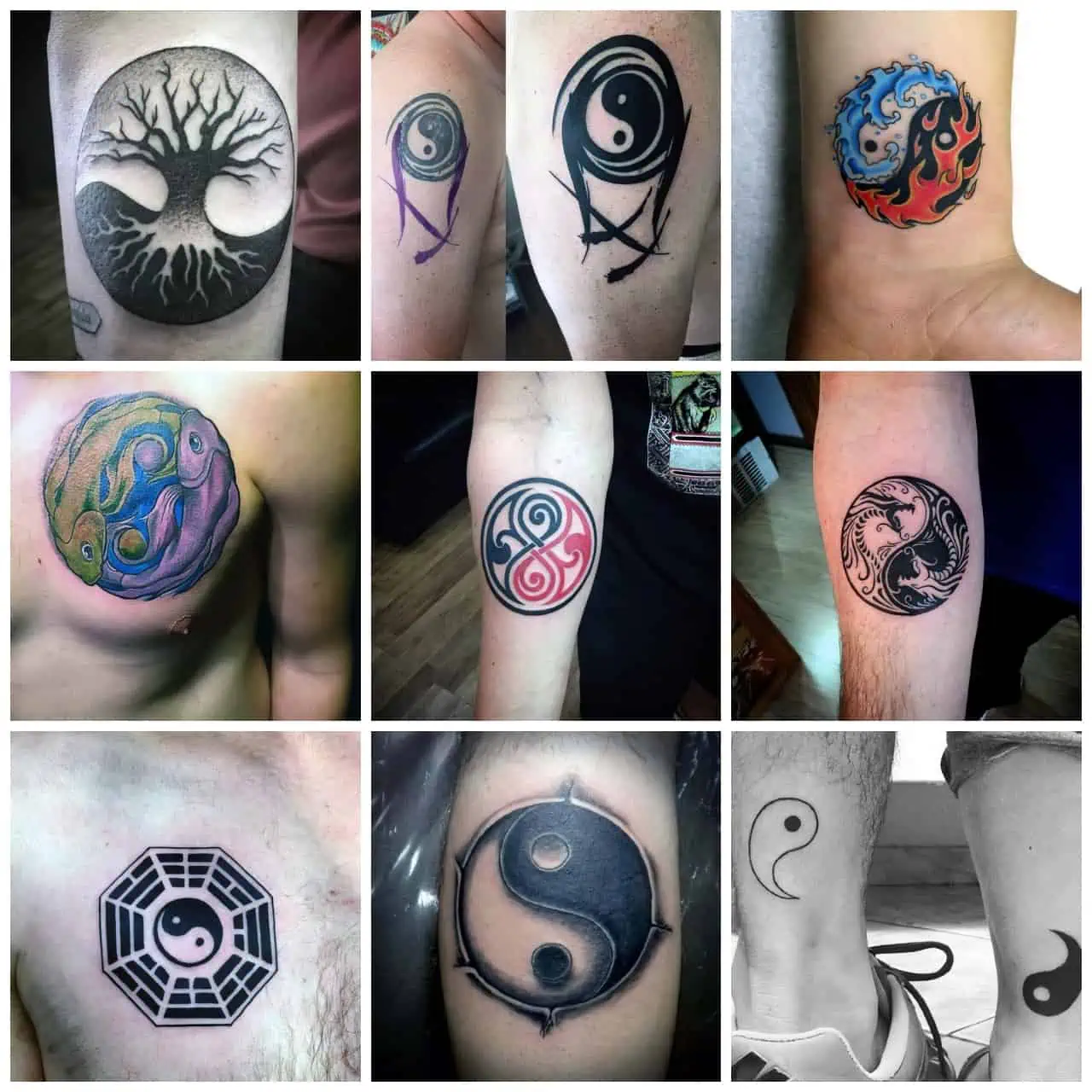This image features a 3x3 grid of nine individual photos showcasing various tattoos, predominantly on arms but also including chest and ankle placements. The top left image depicts a detailed tree tattoo in black ink, showing roots extending into the darker soil with the branches set against a lighter background. Adjacent to it, a tattoo featuring two black swirls, potentially resembling waves or an infinity symbol, appears on either the upper arm or leg. The third tattoo from the left is circular with blue waves on the upper left and orange flames on the bottom, located on an inner wrist.

Moving to the center row, the left image displays a multicolored tattoo of two tropical fish on an arm. The middle photo shows a black and red round figure, likely representing an abstract design, situated on the upper arm. To its right, a tattoo placed on a chest features intricate black and white patterns, forming what might be an octagonal shape.

In the bottom row, the first tattoo on the left illustrates an octagon with alternating black and skin-toned segments. The middle image presents another circular tattoo with contrasting black and skin-toned sections, possibly depicting a figure or pattern within. The final photo in the bottom right corner shows an arm tattoo featuring black teardrops with red dots, positioned next to an ankle tattoo of similar design in black outline.

Finally, this grid also includes an arm with a tattoo tool, resembling a small carving knife, hinting at the tattoo creation process.